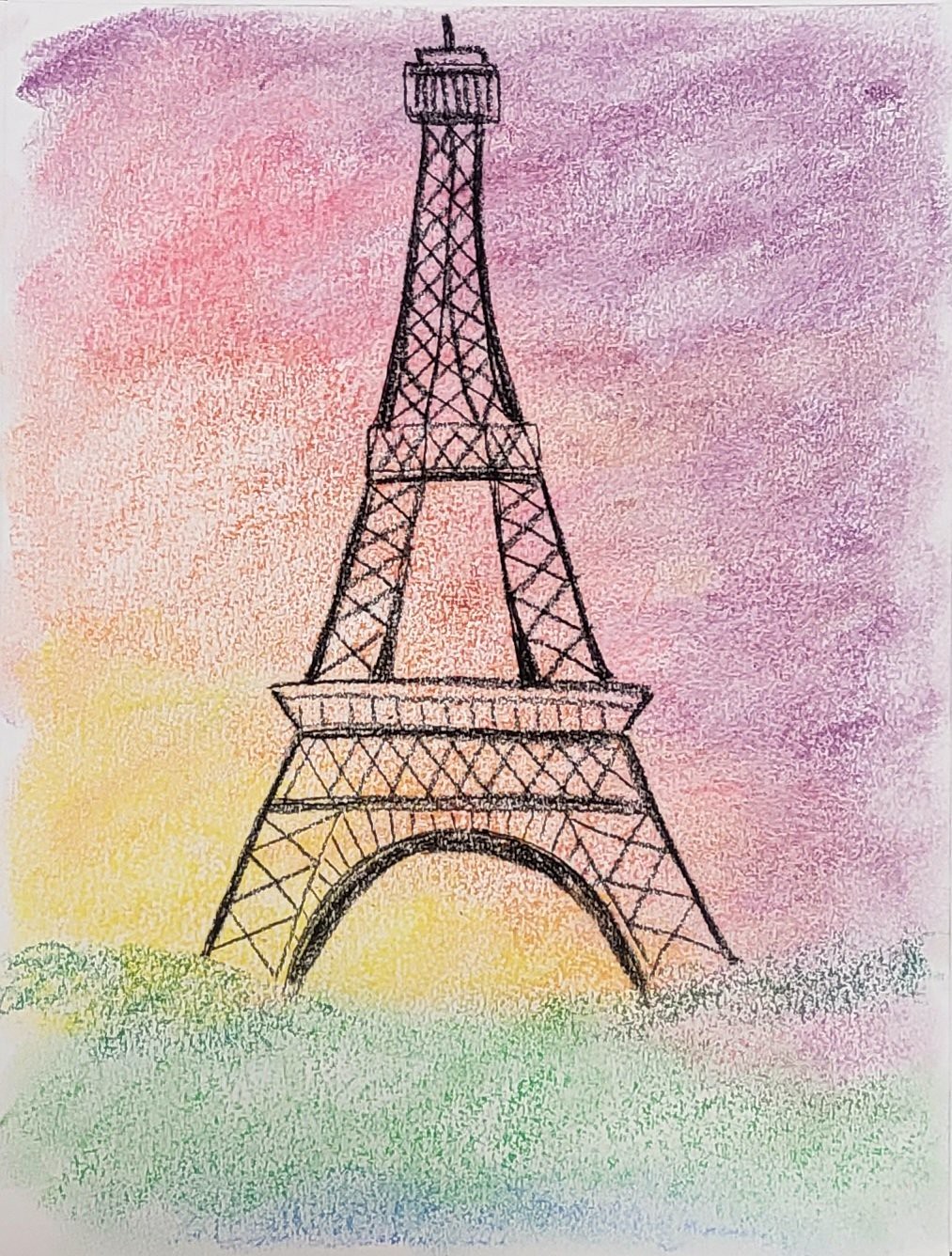A detailed pencil crayon drawing on plain A4 white paper depicts a meticulously rendered Eiffel Tower, outlined in black pencil. The proportions are impressively accurate, suggesting that it might have been created by an older child. The artwork features a gradient background: the upper right corner starts with a deep purple that transitions gradually to an orangey-red hue as it moves leftward behind the Eiffel Tower. The colors shift to a bright yellow at the base, highlighting the two main legs of the prestigious monument. The ground area beneath the Eiffel Tower is shaded in green, suggesting a landscape. This colorful scene conveys the Eiffel Tower against a vibrant sunset, showcasing the young artist's skill in blending and proportion.